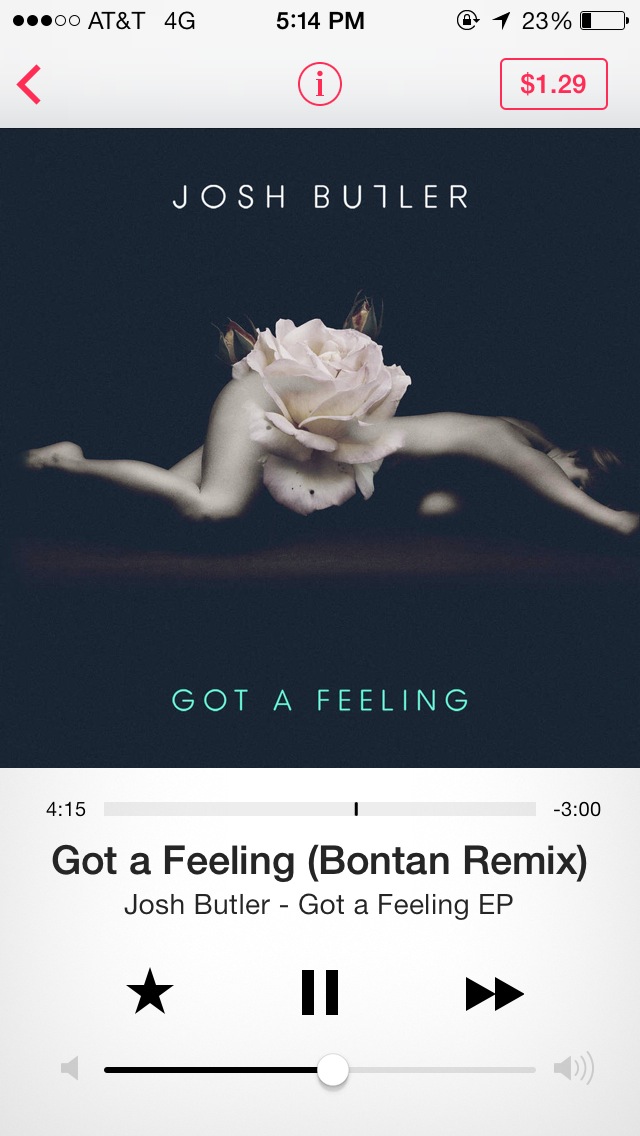The image is a screenshot from a cell phone displaying a music player app for a song available for purchase at $1.29. At the top of the phone screen, it shows the time as 5:14 PM, the carrier AT&T running on 4G, and a battery level of 23%. The song playing is "Got a Feeling (Bonten Remix)" by Josh Butler, from the "Got a Feeling EP". The track has been playing for 4 minutes and 15 seconds, with a progress bar showing 3 minutes remaining. The artwork features a woman lying on a black or brown surface, partially blended into a white flower that conceals her buttocks and private area. The woman's body, facing right, appears to merge with the flower, giving the image an abstract, almost surreal quality. Below the image is the song title "Got a Feeling" in green capital letters, with playback controls and a volume bar beneath it.